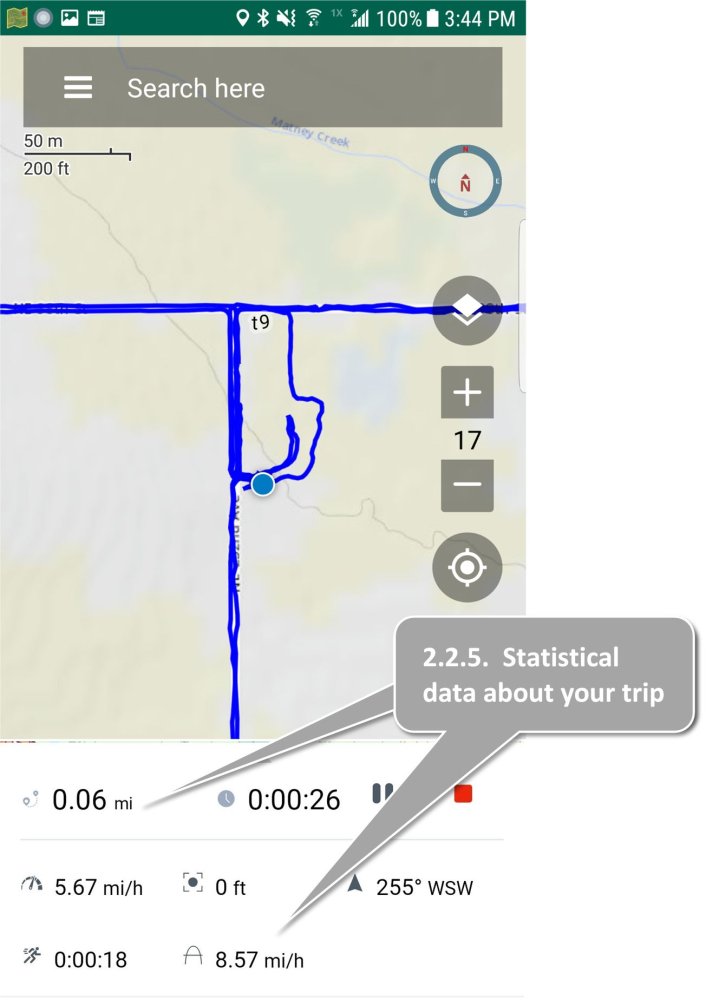The image depicts a smartphone screen primarily displaying a map interface. At the top of the screen, there is a "Search here" text entry section. The central portion of the image is dominated by a detailed map, which includes a compass icon and various settings and options. Notably, a circular blue dot at the map's center indicates the current location of the device. 

Displayed on the screen are several pieces of trip-related information. The device reports a distance of 0.06 miles and indicates that 26 seconds have elapsed. Additionally, there are statistics regarding the vehicle's speed, recorded as 5.67 miles per hour. Various statistical data points relevant to the user's trip are also presented. 

The map itself is crisscrossed with numerous blue lines, likely representing the routes or paths previously traveled by the user. At the very top of the screen, a green status bar provides essential information, including symbols for Bluetooth, Wi-Fi, the current battery percentage, and the time. The background of the map is predominantly white, accentuating the various trip statistics prominently displayed throughout the interface.